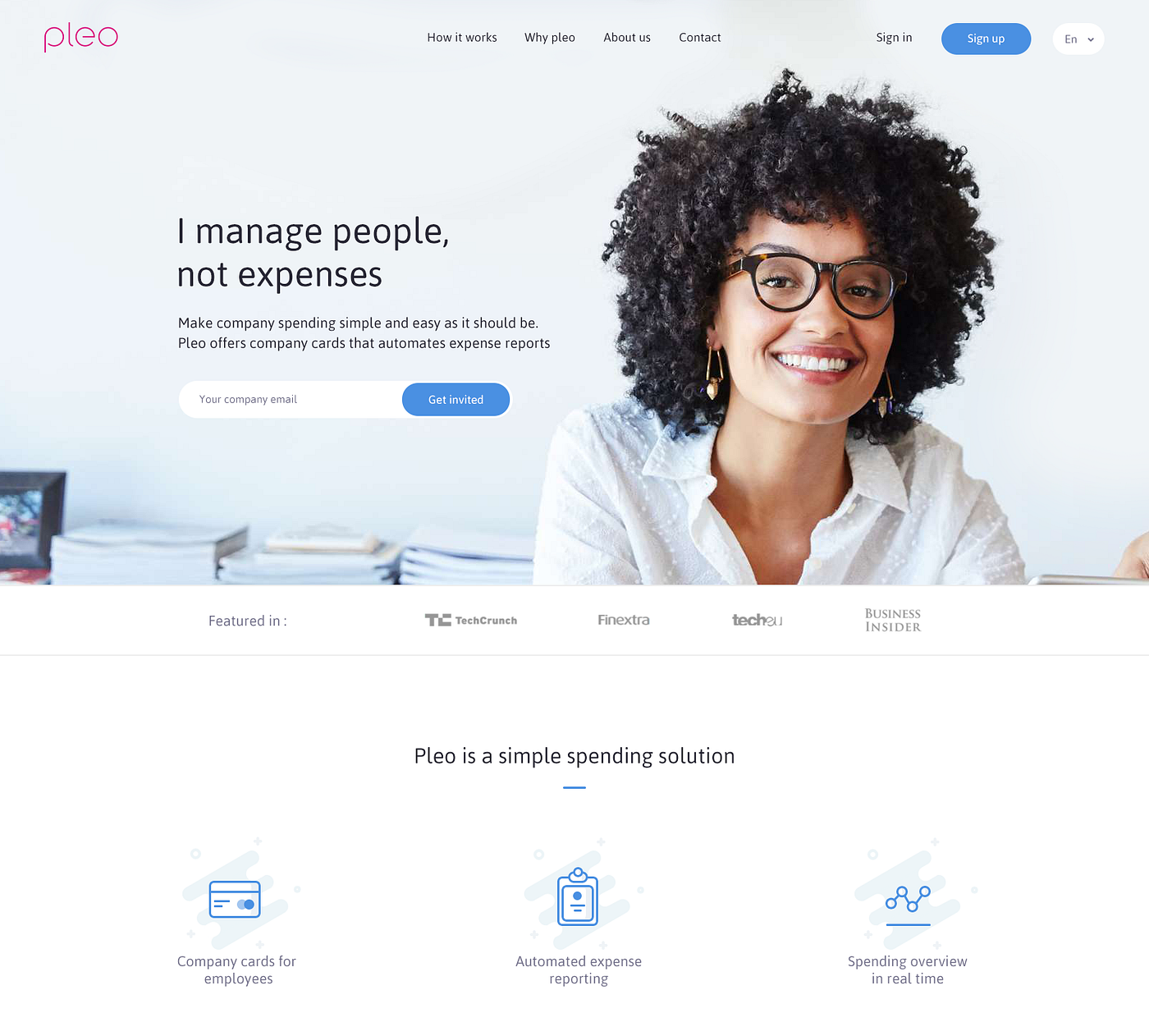The image is a screenshot of a website called Pleo, featuring a sleek interface and a clearly structured layout. The upper left corner prominently displays the Pleo logo, rendered in lowercase red letters against a gray background. Central to the navigation bar are several tabs, including "How It Works," "Why Pleo," "About Us," and "Contact." On the right side of the navigation bar, there are options to sign in, a blue sign-up button, and a dropdown menu labeled "EN."

Dominating the center of the image is a two-column design. On the left, white text reads, "I manage people, not expenses. Make company spending simple and easy as it should be. Pleo offers company cards that automate expense reports." Directly beneath this text is a white input field for entering a company email address, accompanied by a blue button that says "Get Invited."

To the right of the text, there is a photograph of an African American woman with a bright smile, black curly hair, and black glasses. She is dressed in a white button-up shirt and sports dangling, triangle-shaped earrings.

Further down, the bottom left corner of the screen displays a photographic element and three piles of what appears to be paper. Across the bottom of the screen is a tagline: "Pleo is a simple spending solution," followed by three succinct sections. The first section illustrates a credit card, labeled "Company Cards for Employees." The second features an image of a clipboard, with the text "Automated Expense Reporting." The third showcases an icon of lines with circles, titled "Spending Overview in Real Time."